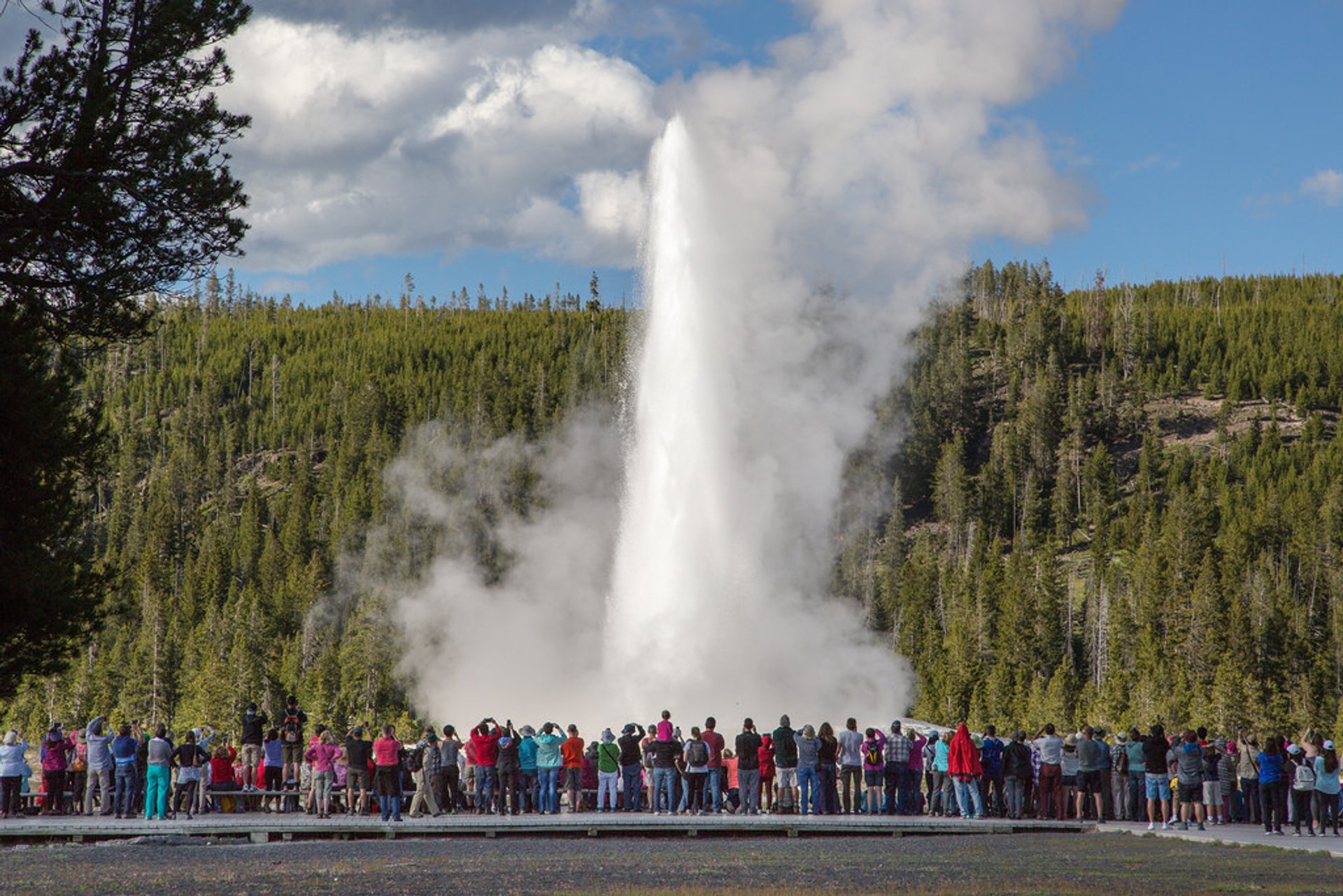This is a detailed photograph captured outdoors in a park or forest, oriented horizontally. The clear blue sky, dotted with clouds, stretches above a small hill densely populated with coniferous trees. The focal point of the image is a geyser, potentially Old Faithful, erupting powerfully, sending white steam and water vapor at least 30 feet into the air, well above the treetops. In the foreground, roughly 100 people in brightly colored outfits are gathered on a viewing platform, standing behind a railing. They are intently watching and photographing the natural spectacle. Yellow flowers add a splash of color to the setting, enhancing the already vivid scene.